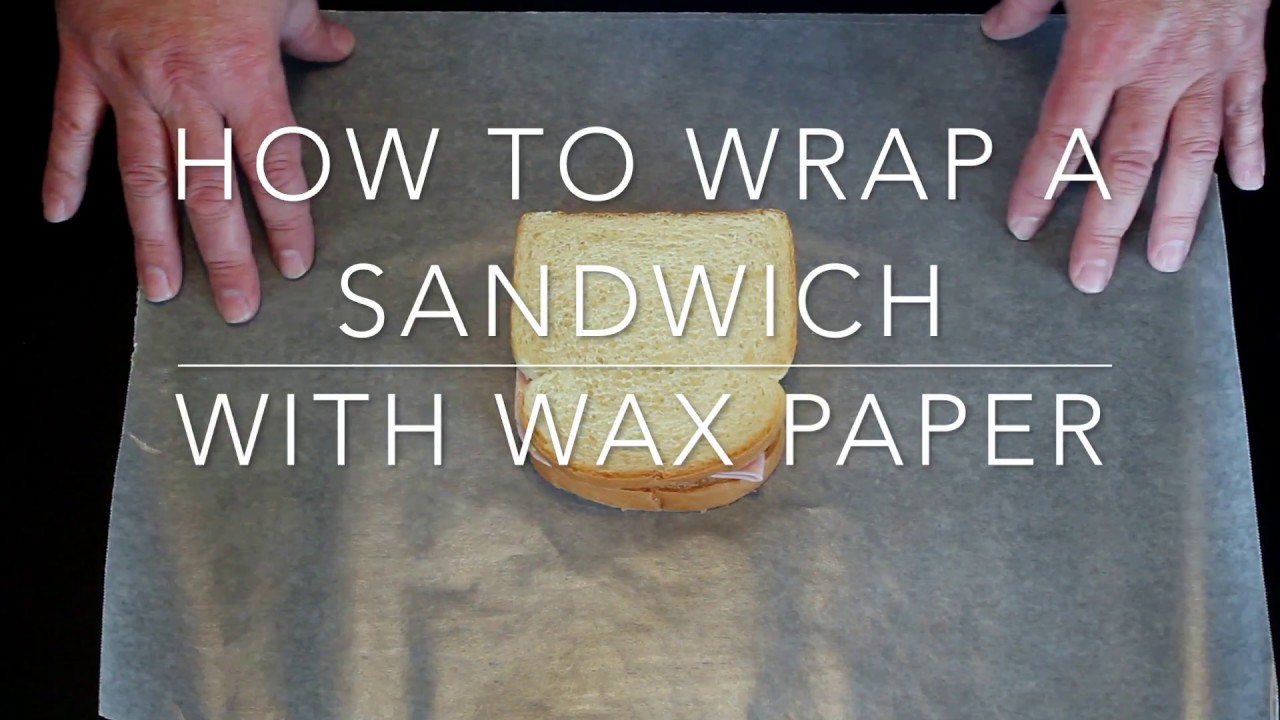The image appears to be a title card or thumbnail for an instructional video titled "HOW TO WRAP A SANDWICH WITH WAX PAPER," with the text displayed in white, all-caps font, possibly featuring a slight drop shadow. The words "sandwich" and "with wax paper" are separated by a thin white horizontal line. The background of the image showcases a piece of wax paper spread out on a dark or black surface. Centered on the wax paper is a sandwich made with slightly yellow potato bread, likely containing meat such as ham or bologna. On either side of the wax paper, a pair of older, weathered, somewhat chubby hands, with slightly red skin, are positioned pressing down on the paper, indicative of the sandwich wrapping process. The overall scene features colors including white, black, beige, brown, and pink, which harmonize to create a focused and practical instructional image.